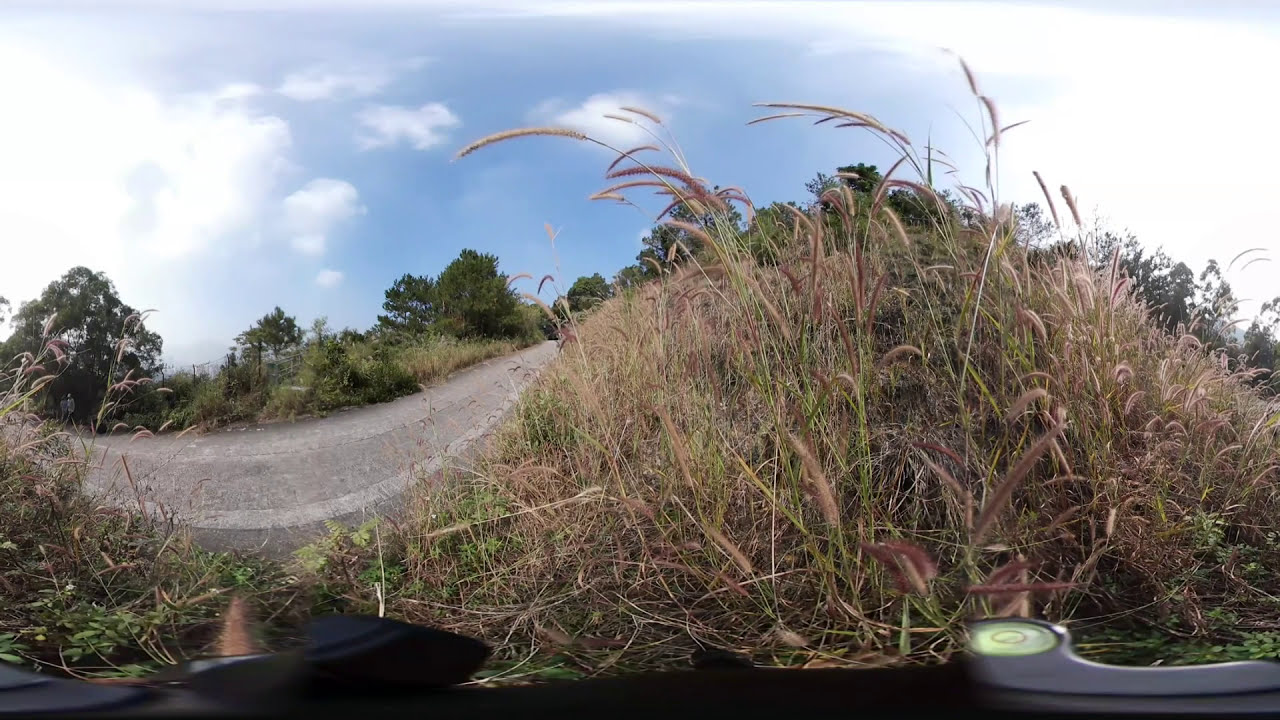The image depicts a close-up view from a very low angle, almost as if the camera is placed directly on the ground, capturing a landscape scene. The foreground is dominated by green and beige blades of grass, interspersed with some brown patches and possibly some wheat-like plants, all on a slight hill. The background reveals a gray road stretching horizontally and forming a hill-like bulge, flanked by thick, green, fluffy-topped trees and assorted vegetation. Above, the sky is a light blue with scattered wispy and puffy white clouds, indicating a clear, sunny day. The image, possibly taken with a GoPro, has a slight distortion, making the road appear as though it's in a bubble. Towards the bottom of the image, an indistinct, horizontally-placed black metal object reflectively catches some of the sky’s light.